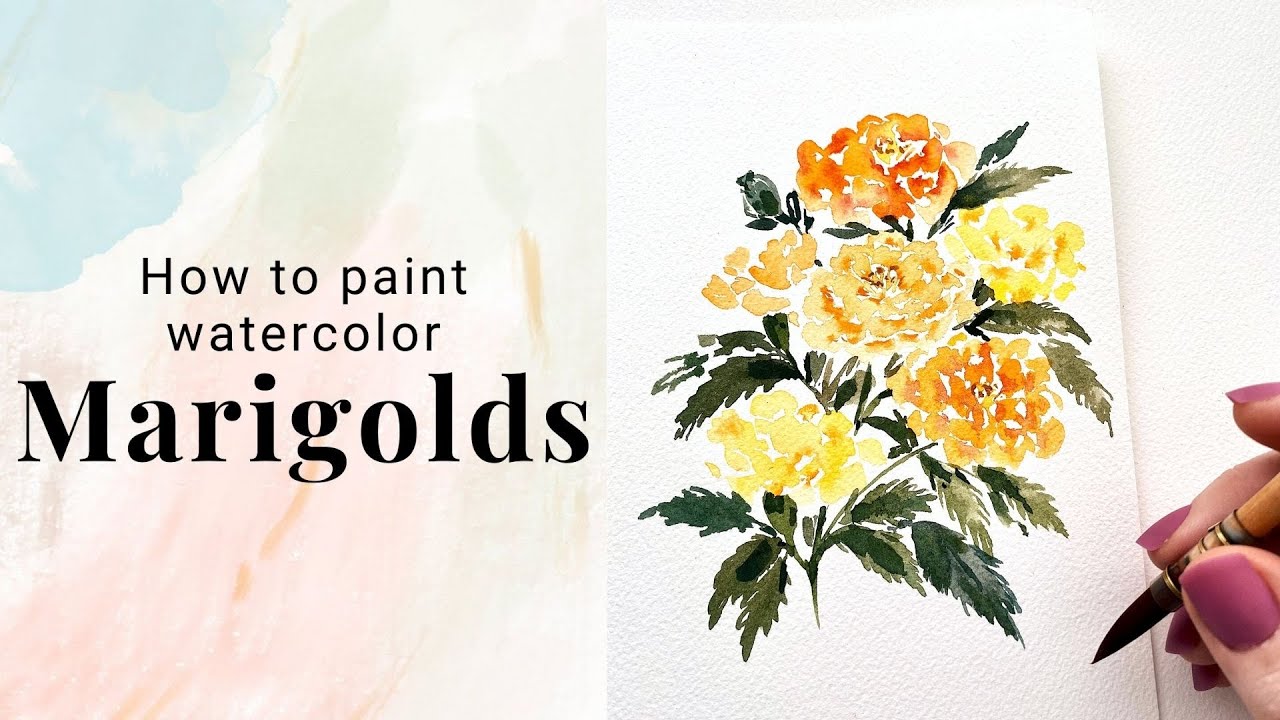The painting titled "How to Paint Watercolor Marigolds" is depicted on a card against a white background. On the left side of the painting, the title is written in black text, with "marigolds" highlighted in bold font. The background around the text transitions from blue at the top left to a bit of sage green in the middle and has soft lines of pink and orange towards the bottom. The right side of the image showcases vibrant orange and yellow marigold flowers with numerous petals and lush, dark green leaves. In the bottom right corner, a woman’s hand, adorned with pink polished nails, is delicately holding a black, sharp-pointed paintbrush, poised over the card.